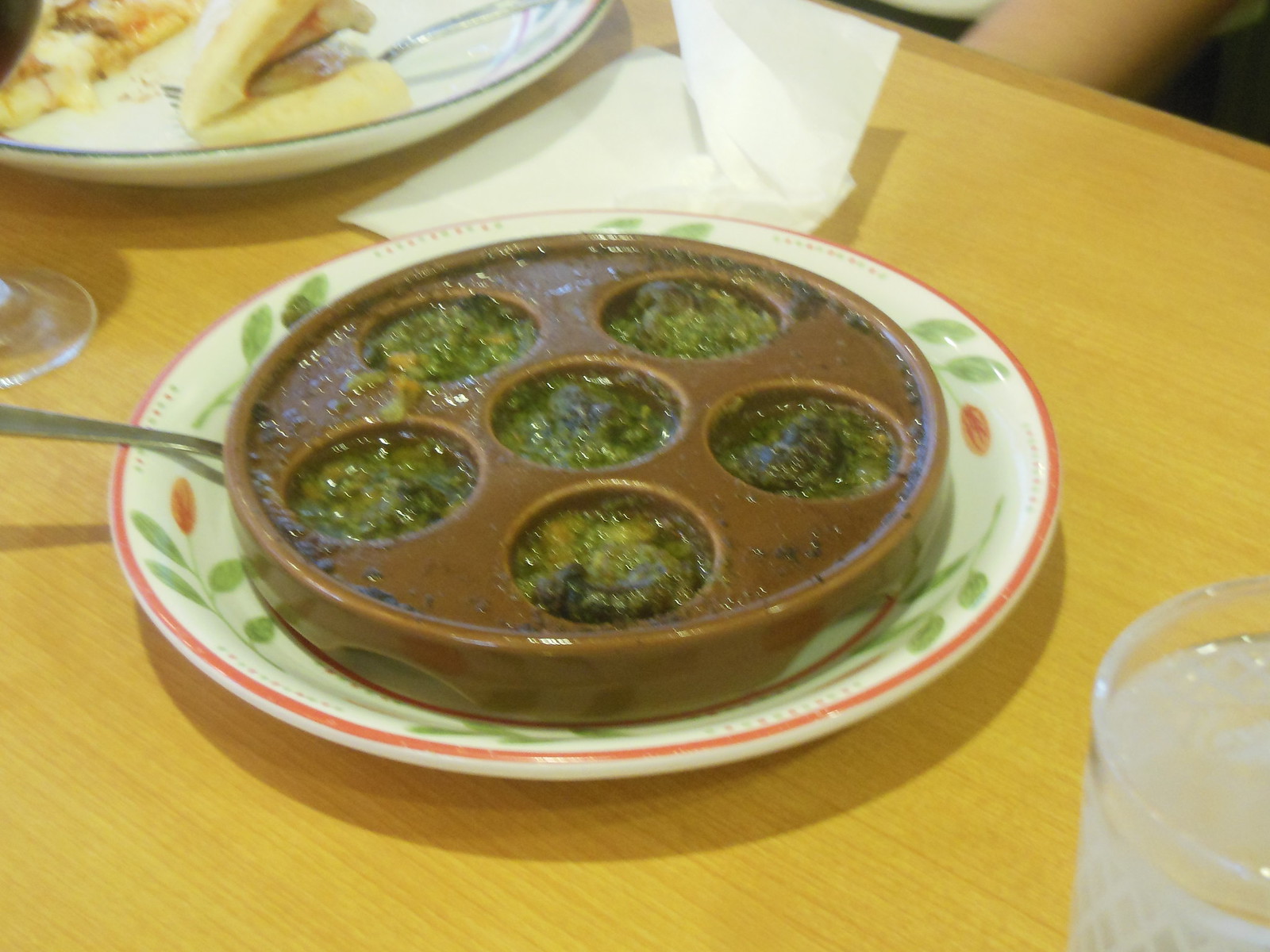The photograph, taken indoors at a restaurant, showcases a detailed and colorful dining setup on a light brown, tan-green wooden table. A white ceramic plate with a decorative red border and a leaf design, featuring what resembles a rosebud on the edge, serves as the base. Atop this plate sits a distinctive, shallow, brownish-orange circular dish featuring six evenly spaced round compartments. Each compartment contains a lumpy green food with hints of brown. To the upper left of the composition, partially visible, are additional elements including a crinkled napkin, a silver spoon, part of a wine glass, and possibly a breaded item or a slice of pizza. The ambiance is further detailed with a glimpse of a person’s arm in the upper right corner, suggesting the presence of diners. Lastly, a glass of water sits in the bottom right, completing the restaurant dining experience.